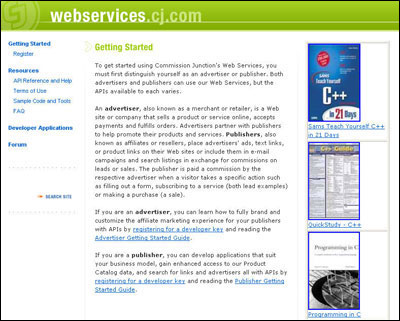The image showcases a web page from the domain "webservices.cj.com," prominently displayed in a lime green header at the top. Beneath this header, the main content area is structured with a clear division to the right of the left margin. 

On the left side, there are several navigation headings for quick access. The heading "Getting Started" is displayed in a blue-colored font, followed by a selection area that is not fully visible. Below this, another heading labeled "Resources" is presented, under which four selectable terms are listed. "Terms of Use" and "FAQ" are legible, while the other two titles remain unclear.

The "Getting Started" section is highlighted in light green and contains a detailed paragraph of approximately four lines. Following this is the main body content, where the word "appetizer" stands out in bold and is also repeated in a subsequent paragraph consisting of four lines. This paragraph includes highlighted elements in sky blue font, which are underlined and likely clickable links. Another brief paragraph with similar formatting follows.

On the right side of the page, there are three images, one of which depicts the C++ programming language. This layout creates an organized and navigable interface, with important sections emphasized through color and formatting variations.